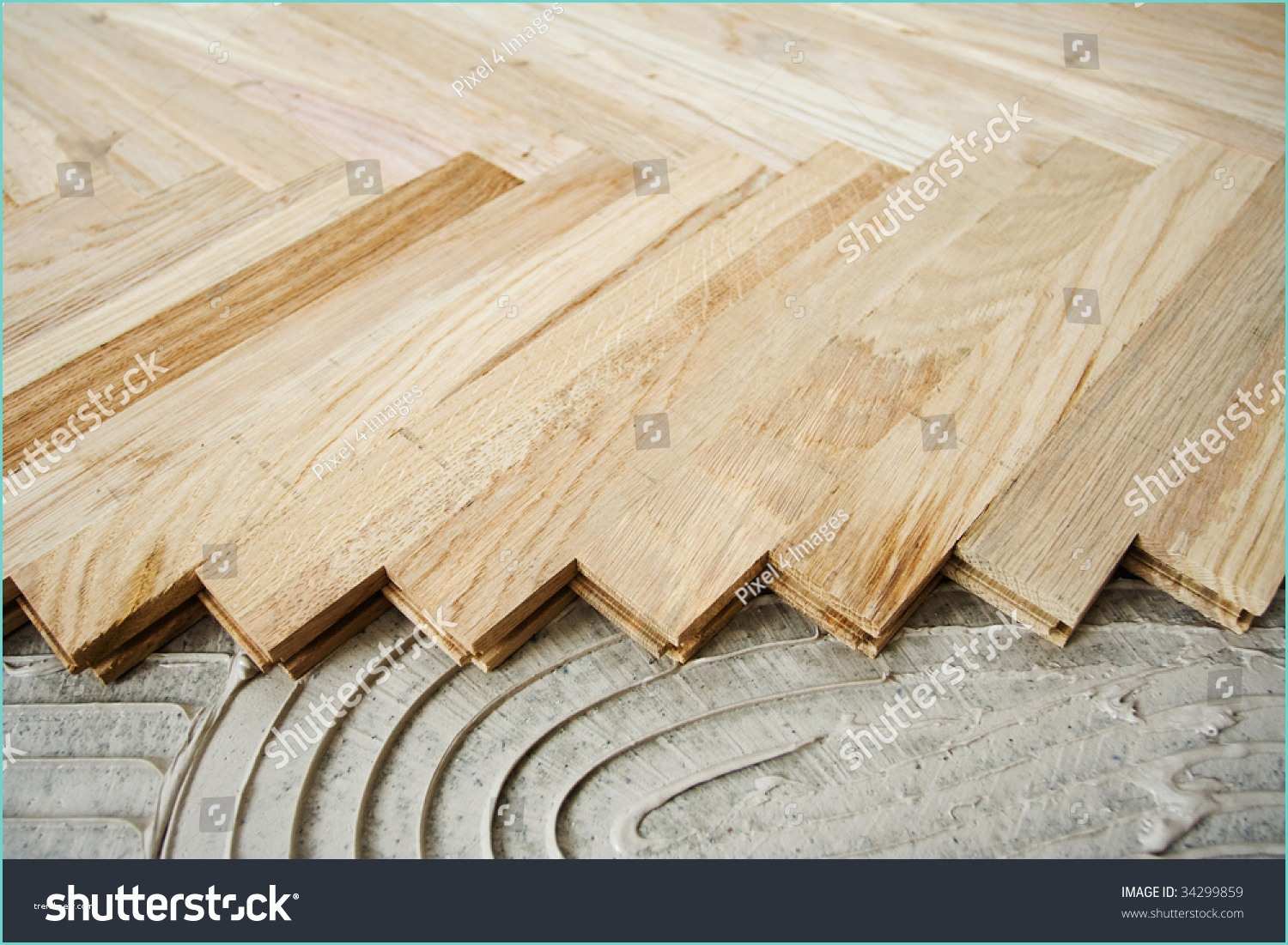This image is a Shutterstock stock photo depicting an incomplete flooring project with rectangular pieces of unfinished, light-colored wood. The wooden beams are aligned in a jagged, up-and-down pattern, creating a series of 90-degree angles where the beams meet. At the bottom of the image, there's a visible section of the underlying surface, likely cement or another gray, hard material, with adhesive patterns in both circular and horizontal lines. The overall color palette includes beige, brown, gray, dark gray, tan, and white. Watermarks, including the word "Shutterstock" in a diagonal, white font and cropping icons, are spread across the image. Additionally, the bottom right corner displays "image ID 34299859" and "www.shutterstock.com." The photograph is oriented as a horizontal rectangle and showcases an indoor style typical of a construction flooring project.